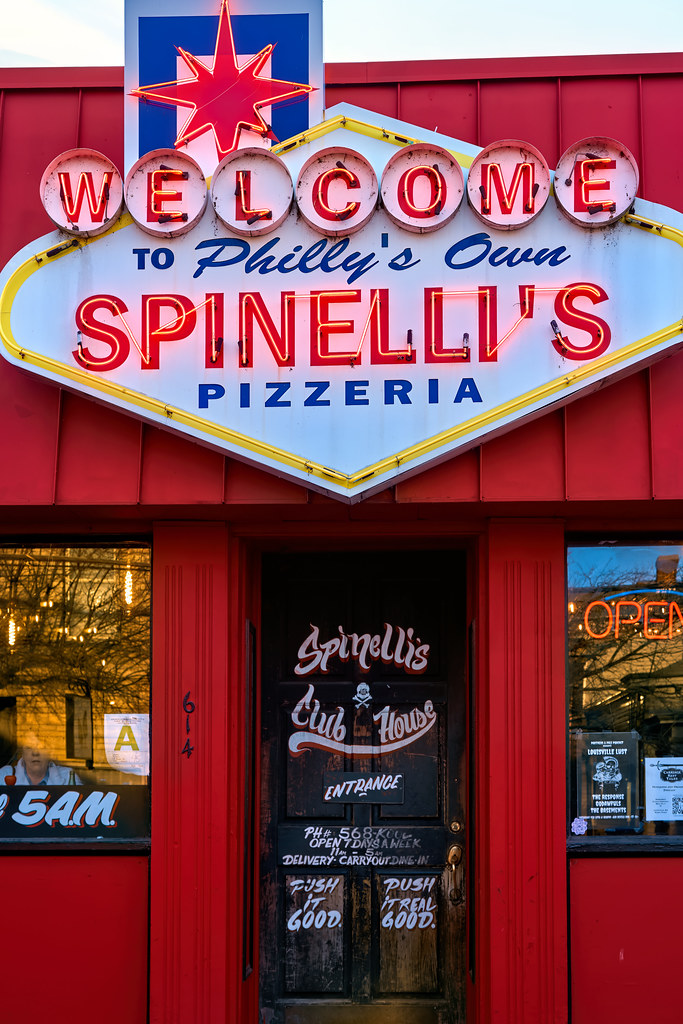The image depicts a color photograph taken in daylight of the storefront of "Spinelli's Pizzeria," an intriguing establishment housed in a red metal building that gives off an old-style vibe. Dominating the scene is a large, attention-grabbing sign reminiscent of the "Welcome to Las Vegas" marquee. This stunning sign features a lit-up red starburst on the upper left and is adorned with neon lights throughout. 

The sign conveys a welcoming message in a tiered format: "Welcome" in vibrant red neon; "To Philly's Own" in blue text; "Spinelli's" illuminated in red neon; and "Pizzeria" below in blue text. All this signage is set against a pristine white background.

Beneath this prominent sign is a black door, its paint visibly weathered and worn, which serves as the entrance to "Spinelli's Clubhouse." An artistic and flowing script on the door reads "Spinelli's Clubhouse" with a skull and crossbones motif. Also inscribed are various details including "Entrance," the phone number "PH 568 KOOL," and operation hours "Open seven days a week, 11 a.m. to 5 a.m." Additional directives on the lower panels state "Push It Good, Push It Real Good."

Flanking the door are large plate glass windows. To the right, a partially illuminated "Open" sign flickers, while on the left, an 'A' health grade notice is prominently posted in the window, echoing the establishment's commitment to quality. Through this left window, the reflection makes viewing difficult, but you can discern a person inside, clad in a white jacket, possibly a staff member ready to serve.

The overall scene is one of vibrant activity and inviting design details, promising an engaging dining experience at "Spinelli's Pizzeria."